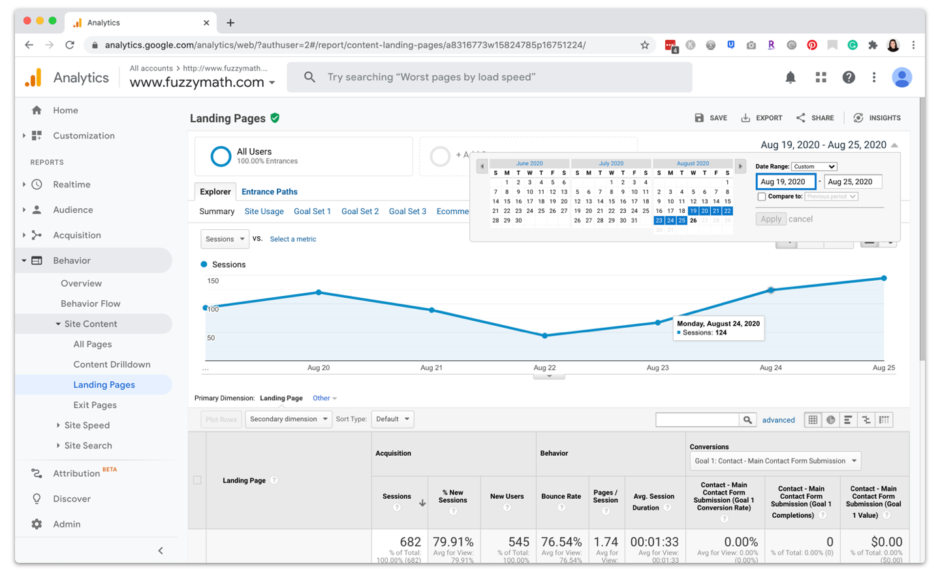This image is a screenshot from Google Analytics, accessible via the URL analytics.google.com. It provides a detailed look at the various sections of the Google Analytics interface, including navigation menus such as Home, Customization, Reports, Real-Time, Audience, Acquisition, Behavior, and Discover. Highlighted within the Behavior section are subcategories like Overview, Behavior Flow, Site Content, Site Speed, Site Search, and Attribution.

The focal point of the screenshot is the Behavior Flow segment for the website www.fuzzymath.com, specifically analyzing landing pages. The data displayed is filtered to show all users and indicates that 100% of entrances are through landing pages. The explorer view offers various tabs such as Summary, Site Usage, Goal Set 1, Goal Set 2, and Goal Set 3. The primary dimension set is Landing Page, with an additional secondary dimension also labeled Landing Page.

Key metrics highlighted include the number of sessions (682) and the percentage of new sessions (9.91%). This screenshot encapsulates comprehensive analytical data, enabling a thorough understanding of user behavior and site performance.